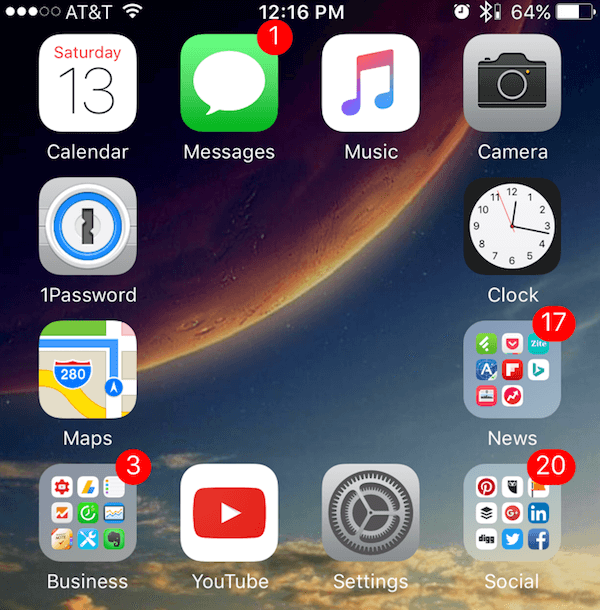This image captures a portion of a device screen, possibly from a tablet, cell phone, or computer. The screen displays an array of square icons arranged in a grid pattern, enclosing an empty center space. Each icon features a small image related to its function, with its corresponding name written in white text beneath it. The background of the image exhibits a beautiful gradient starting from the top-left corner, depicting a partial moon in a golden yellow hue that transitions into a brownish-red and eventually a dark area. Moving towards the center, the background shifts to a light blue or darker blue sky adorned with light gray to white clouds, illuminated by sunlight.

At the very top, the carrier "AT&T" and the current time "12:16 p.m." are displayed in white text, centered perfectly. The battery icon, located at the top right corner, shows a charge of 64%. Notably, the center of the icon grid remains clear, offering an unobstructed view of the moon against the sky background.

Amongst the icons, the "Messages" icon stands out with a red notification circle in the top right corner, indicating one unread message. The icon is green with a white speech bubble in its center. The overall composition of the screen is visually appealing, balancing functionality with the aesthetic beauty of the background.